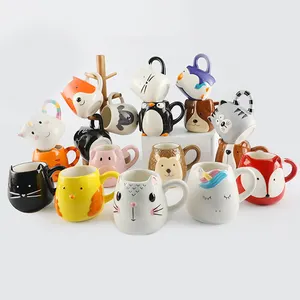This image captures a vibrant and whimsical collection of approximately 18 ceramic coffee mugs, each portraying charming animal characters. The assortment includes black cats, colorful birds, penguins, dogs, unicorns, foxes, raccoons, hedgehogs, pigs, and sheep. The mugs are distinct in their appearances, featuring varied faces, whiskers, eyes, and a spectrum of colors including yellow, white, red, black, pink, brown, and blue. They are arranged creatively: three hang from a wooden mug tree, four sit atop a white box, and several others are perched on one another in a diagonal fashion to maximize space. The entire collection faces the photographer, offering an endearing display of animated expressions and playful charm.